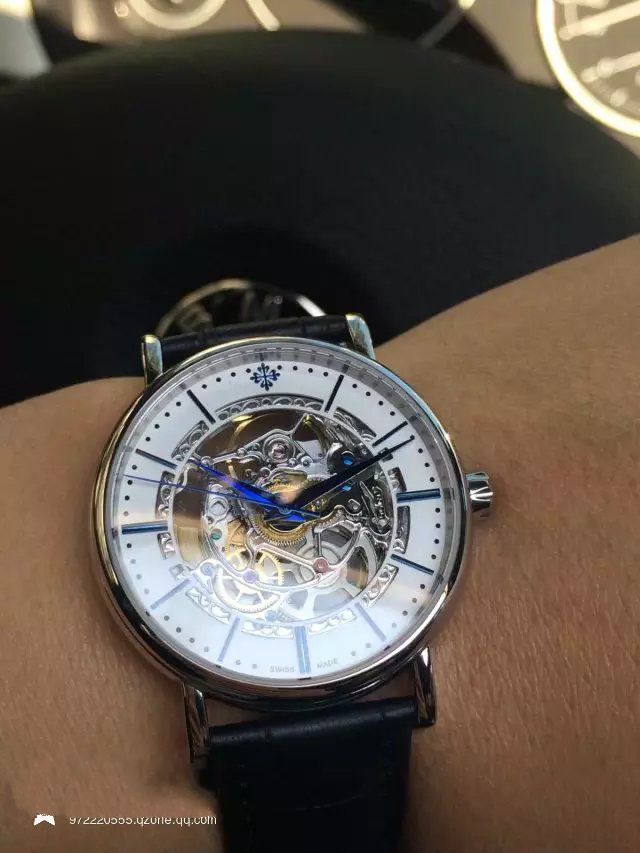This color photograph features a close-up of a wrist adorned with an intricate, steampunk-inspired watch. The black leather band of the watch is prominently visible on both the top and bottom of the wrist. The large, round dial is centrally located in the lower portion of the image, with a silver time-setting knob on its right side. The dial showcases a complex design, reminiscent of anime art, with visible silver and gold gears and inner workings. The watch face has a silver rim, bordered by a white ring marked with lines for hours and dots for minutes, although there are no numerical values. The minute hand is a striking blue, while the hour hand is black, indicating the time as 10:11. The background is a black blur with no discernible details, and there is white text and a logo or signature in the bottom left-hand corner, adding to the sophisticated aesthetic of the watch.